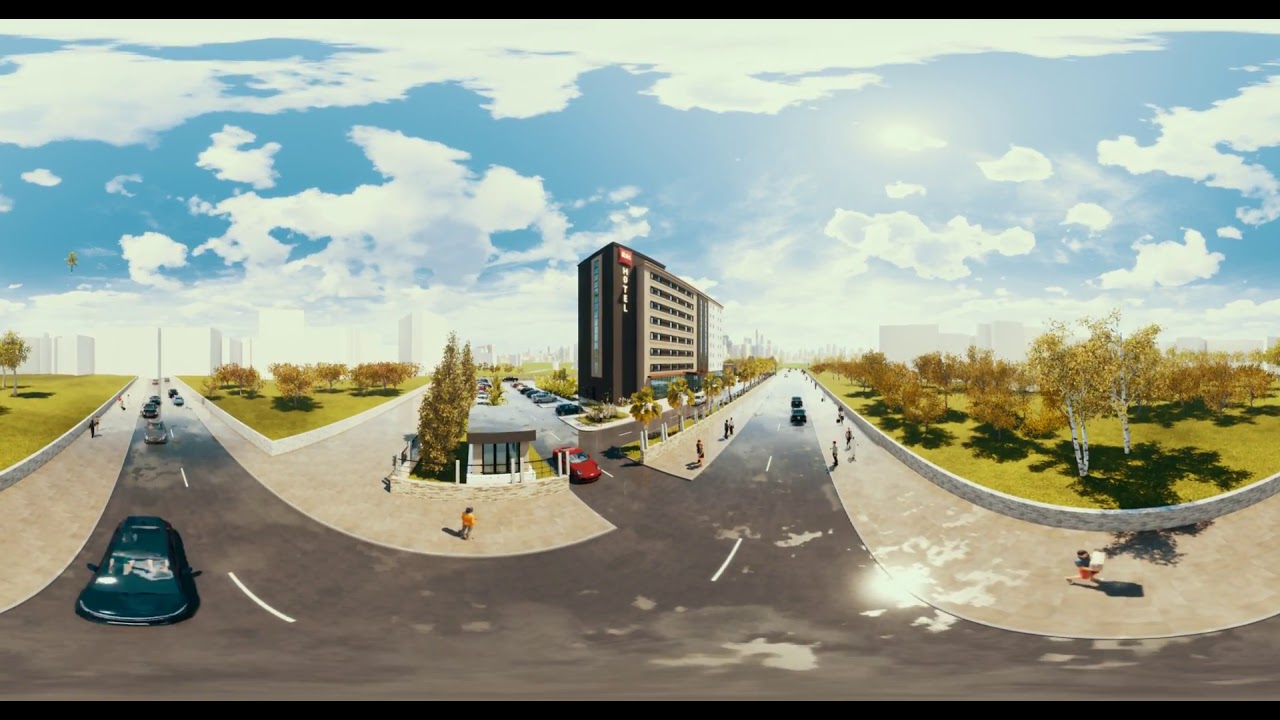This image is an intricate 3D artist's rendering of a vibrant vacation resort or hotel set in a stylized, almost surreal landscape. The central focus is a multi-story hotel, prominently featuring a vertical sign with the word "hotel" on its dark facade, contrasted by a lighter facade adorned with numerous windows. The hotel is surrounded by various elements that blend urban and natural settings.

In the foreground, a stylish dark automobile is seen driving towards the bottom of the frame on a curved street, while a small gatehouse stands nearby. Adjacent to the hotel, a road curves around and stretches off into the distant horizon, illuminated by bright sunlight reflecting on the highway. The image also showcases a parkland area to the right, featuring trees with brown leaves, enhancing the autumnal feel. Various roads intersect throughout the scene, with numerous cars and people either walking on the sidewalks or through a busy parking lot, emphasizing the area's lively atmosphere.

The backdrop includes stylized, mock-up white buildings creating the impression of a distant city or suburb. The sky is artistically rendered with multiple types of clouds and bright sunlight emerging in the upper right portion of the image. This vibrant, highly detailed illustration, although artificial, successfully conveys the essence of a middle to upper-class vacation spot, set in a picturesque, outdoor suburban or urban environment with an abundance of greenery and fall colors.